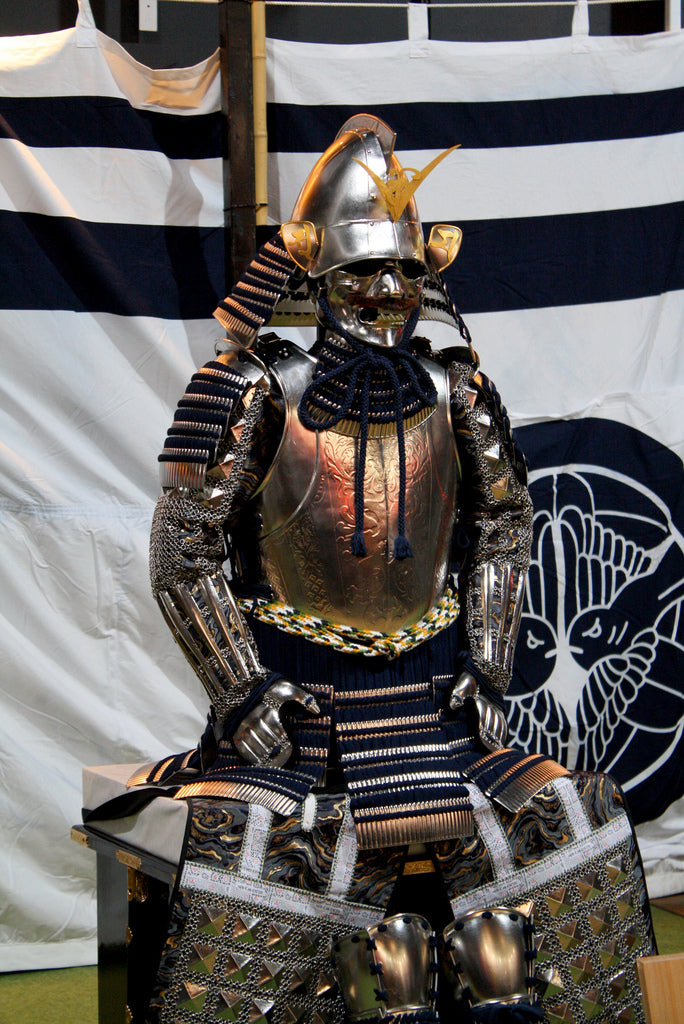This color photograph captures an elaborate, futuristic suit of armor reminiscent of the Tin Man from "The Wizard of Oz." The armor is a blend of silver and gold with a highly reflective finish. The figure's face is obscured by a silver mask, appearing dark and inscrutable beneath a helmet adorned with a gold emblem. The suit features a grimacing face mask, a breastplate with a cord around the neck, and iron mesh sleeves that integrate decorative metalwork, extending down to gauntlets and leg protectors. The ensemble may either conceal a person or stand as a remarkably detailed mannequin. In the background, a black and white flag with a black medallion depicting two birds adds to the scene's atmosphere, reflecting orange lights that illuminate the vest area of the armor. The figure is standing tall, possibly propped on a bench or table, lending an air of solemnity and intrigue to the entire composition.